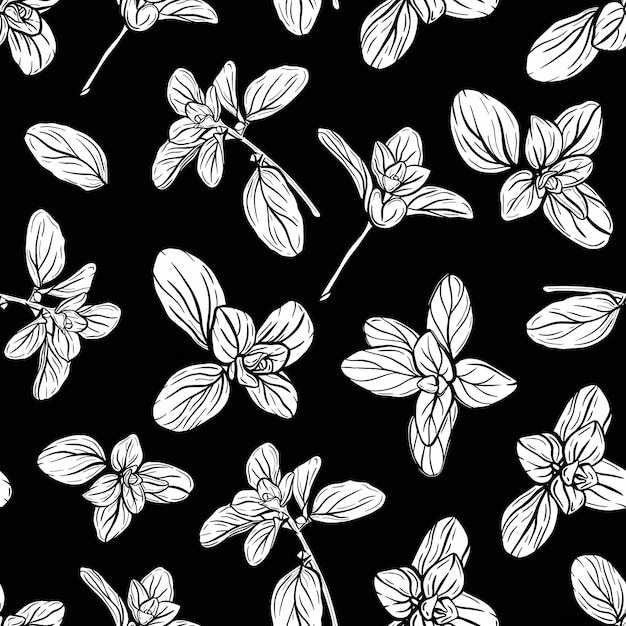This black-and-white image features a captivating hand-drawn pattern of medium-sized flowers set against a black background. The illustration, likely created using a digital painting application such as MS Paint, showcases a repetitive design suitable for fabrics or paper products. The flowers, which all appear to be of the same species, possess five to six oval-shaped petals and are depicted without buds at their centers. Some flowers are attached to short, two to three-inch long stems, while others are standalone, floating in space. The leaves within the design are intricately detailed with vein-like structures, appearing in various directions and enhancing the complexity of the pattern. The arrangement of flowers offers diverse perspectives, with some viewed from above and others in profile. The overall composition is devoid of any text or framing, concentrating purely on the exquisite floral line art.